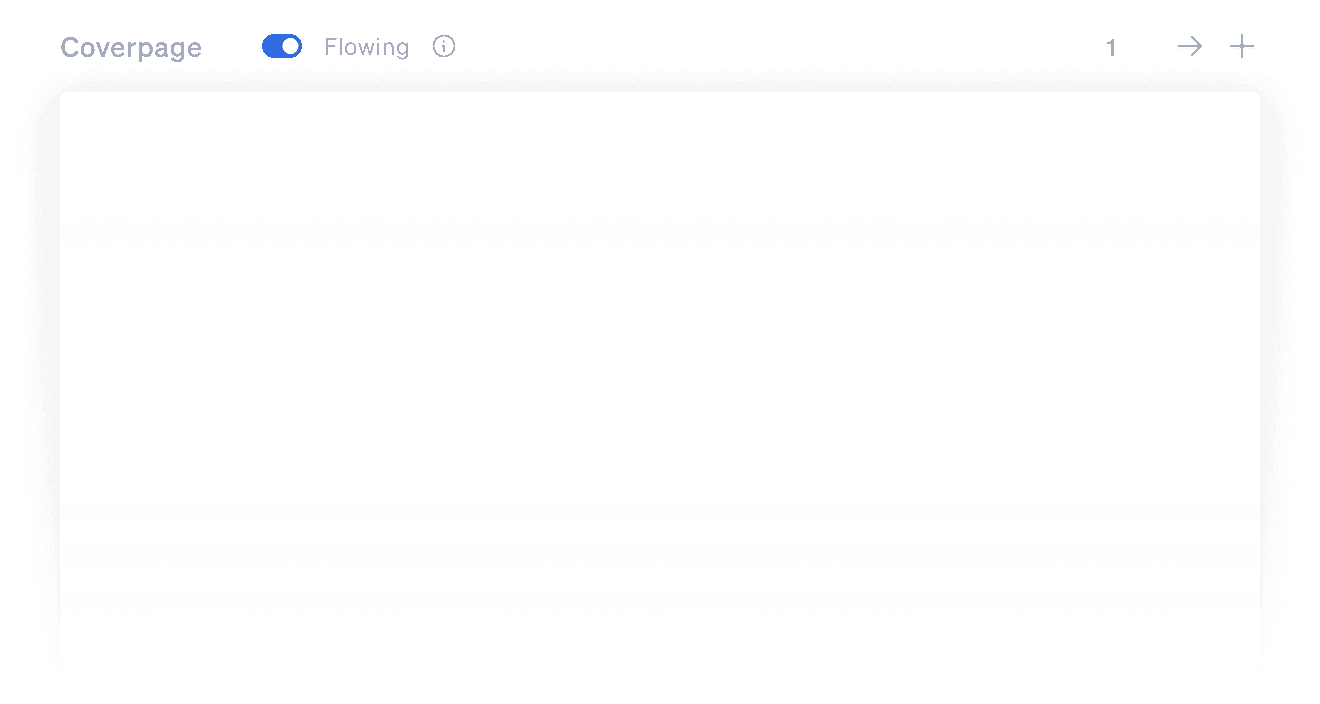The image features a design interface with several distinct elements. In the top left corner, grey text prominently displays the term "Cover Page." Below this, a blue pill-shaped icon with a circle inside indicates that the toggle switch is on, with the toggle positioned to the right. Adjacent to this icon, the word "FLOW" is written in unembellished text. 

Next to "FLOW" is an eye icon enclosed within a circle. On the right side of this section, there is a sequence of symbols: a plus sign, followed by an arrow pointing right, and a numerical "1." The arrow points towards the plus sign, while the number "1" is situated to the left of the arrow.

The main section of the image, occupying approximately 80% of the frame, is predominantly white with a subtle grey shadowing effect, adding depth to an otherwise blank space.